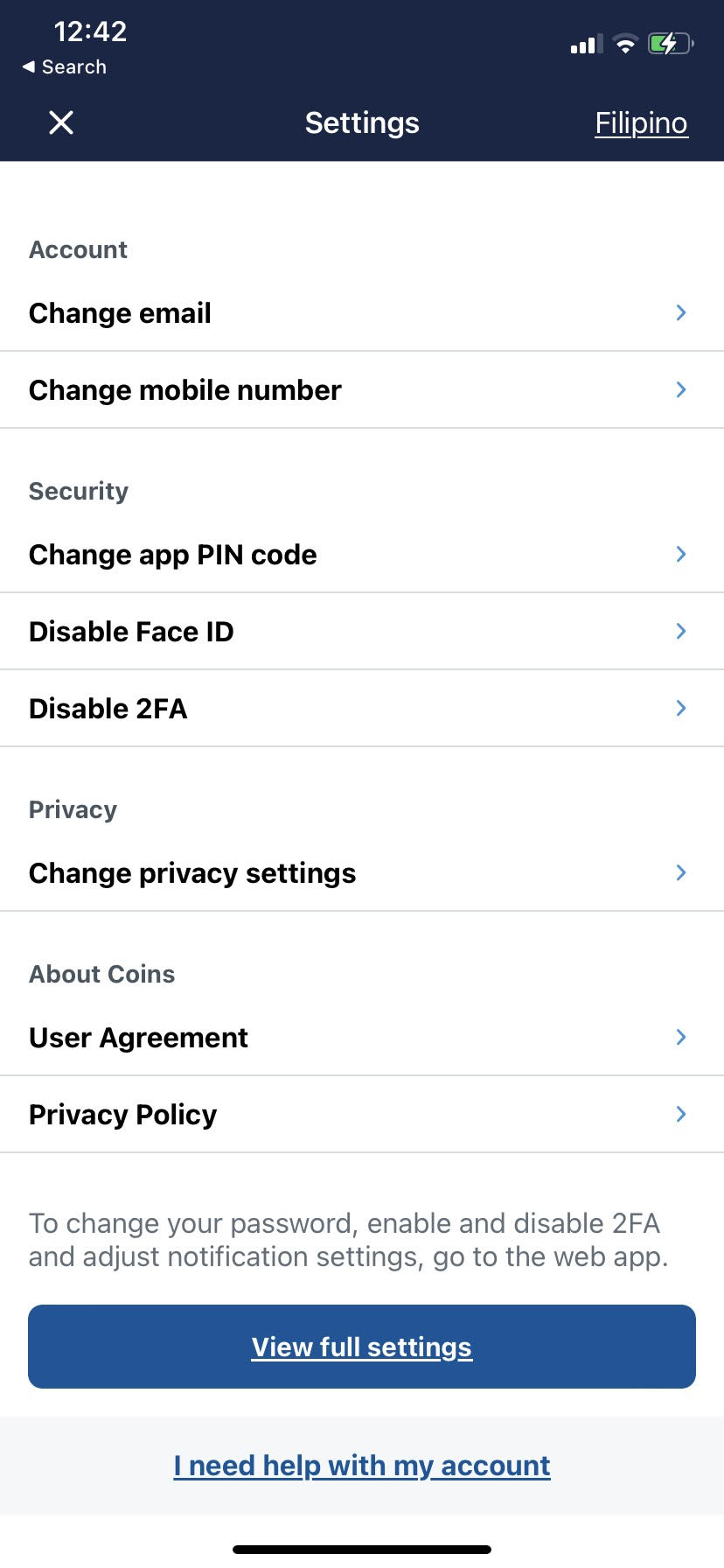A screenshot captured from a mobile phone displays several interface elements. At the very top, there is a navy blue status bar showing the time as 12:42. The battery icon is half full and charging, indicated by a thunderbolt symbol. Next to it, Wi-Fi and mobile signal icons are visible. Below the status bar, the screen shows the "Settings" menu with "Filipino" selected and underlined in white.

The main content is comprised of a white page segmented into several sections. At the top, in gray font, it says "Account." This section includes "Change Email" with a right-pointing arrow, and "Change Mobile Number" also with a right-pointing arrow.

Next, under the "Security" section, the options "Change App PIN Code," "Disable Face ID," and "Disable 2FA" each have arrows pointing to the right. 

Following this, the "Privacy" section is labeled in gray font, with the option "Change Privacy Settings" available underneath in black font, followed by a right-pointing arrow.

The final section, labeled "About Coins" in gray font, includes "User Agreement" and "Privacy Policy," each accompanied by a right-pointing arrow. 

At the bottom, a note informs users that to change passwords, enable or disable 2FA, and adjust notification settings, they need to access the web app.